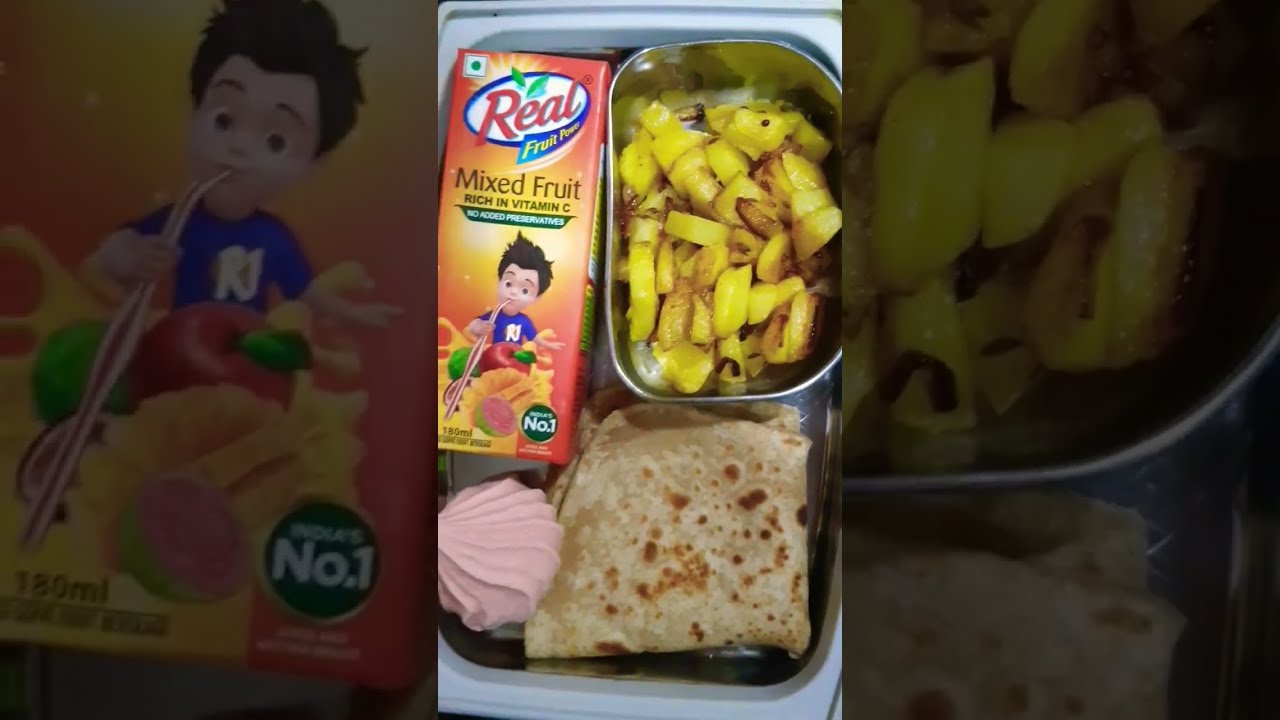The image depicts a close-up of a child's school lunch tray. In the upper left-hand corner, there's a juice box labeled "Real Fruit Power, Mixed Fruit, and Vitamin C" with a cartoon boy drinking through a straw. To the right of the juice box, a small metal container holds what appears to be brown-edged yellow fruit, likely peaches or pineapples. Below the juice box is a folded tortilla or flatbread, and to its right lies a small pink meringue cookie with a dollop shape and lined texture. All items are arranged within a metallic tray that fits snugly inside a white plastic frame, giving an organized and compartmentalized view of the lunch components.